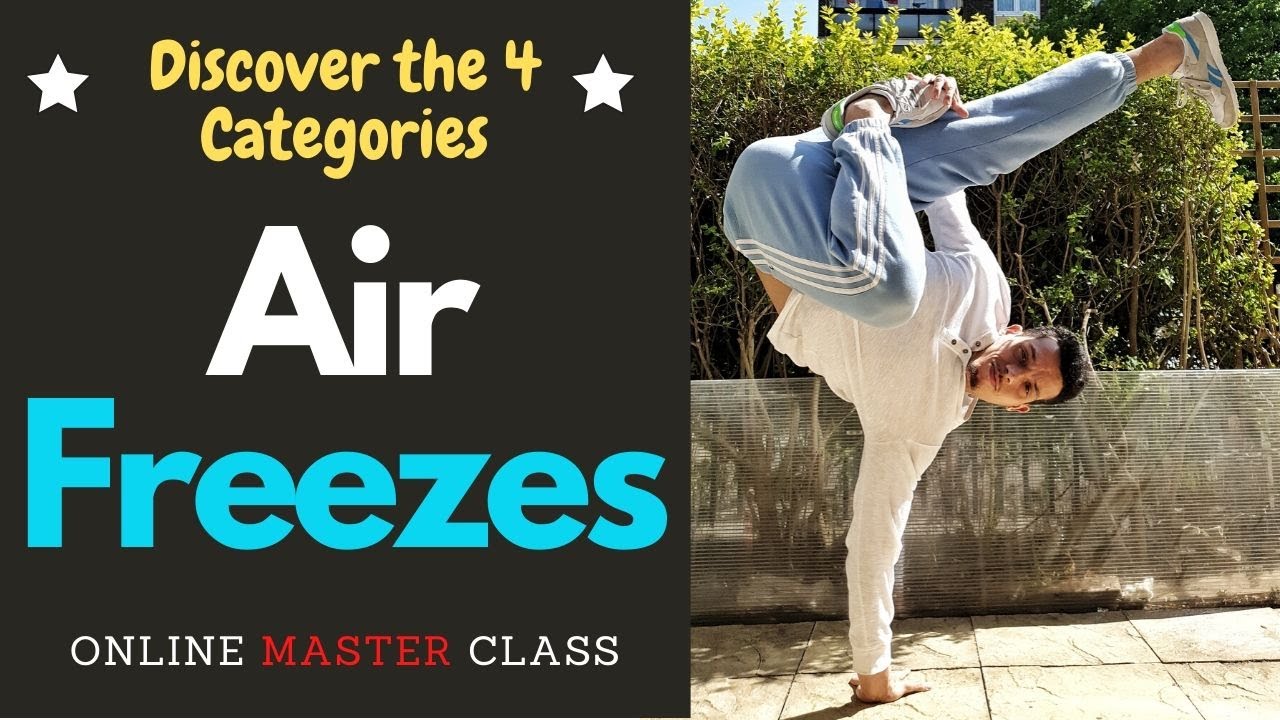In this colorful, portrait-oriented photograph, a young man is captured mid-breakdance, performing an impressive one-handed handstand. The man, who appears to be in his late 20s, has dark skin, black hair, and a goatee, and he is smiling directly at the camera. He is dressed in a cream-colored long-sleeve shirt, blue track pants with white stripes down the sides, and white and grey shoes with blue and grey highlights. His left hand is firmly planted on a concrete block path, holding his entire body aloft, while his right leg extends straight out to the side and his left leg is bent, with his right hand grasping his foot behind his leg. His head is tilted sideways, parallel to the ground.

The background features a white mesh fence with green shrubs, some trees, and what appears to be a wooden fence and a building, hinting at a sunny outdoor setting.

The left side of the image is occupied by a black square with vibrant text. At the top of the square, in yellow letters and flanked by white stars, is the phrase "Discover the Four Categories." Below this, the word "Air" is prominently displayed in white text, followed by the word "Freezes" in bold blue letters. At the bottom of the square, the phrase "Online Master Class" is written, with "Master" in red and "Online Class" in white. The combination of photographic realism and graphic design elements creates a striking and dynamic visual presentation.